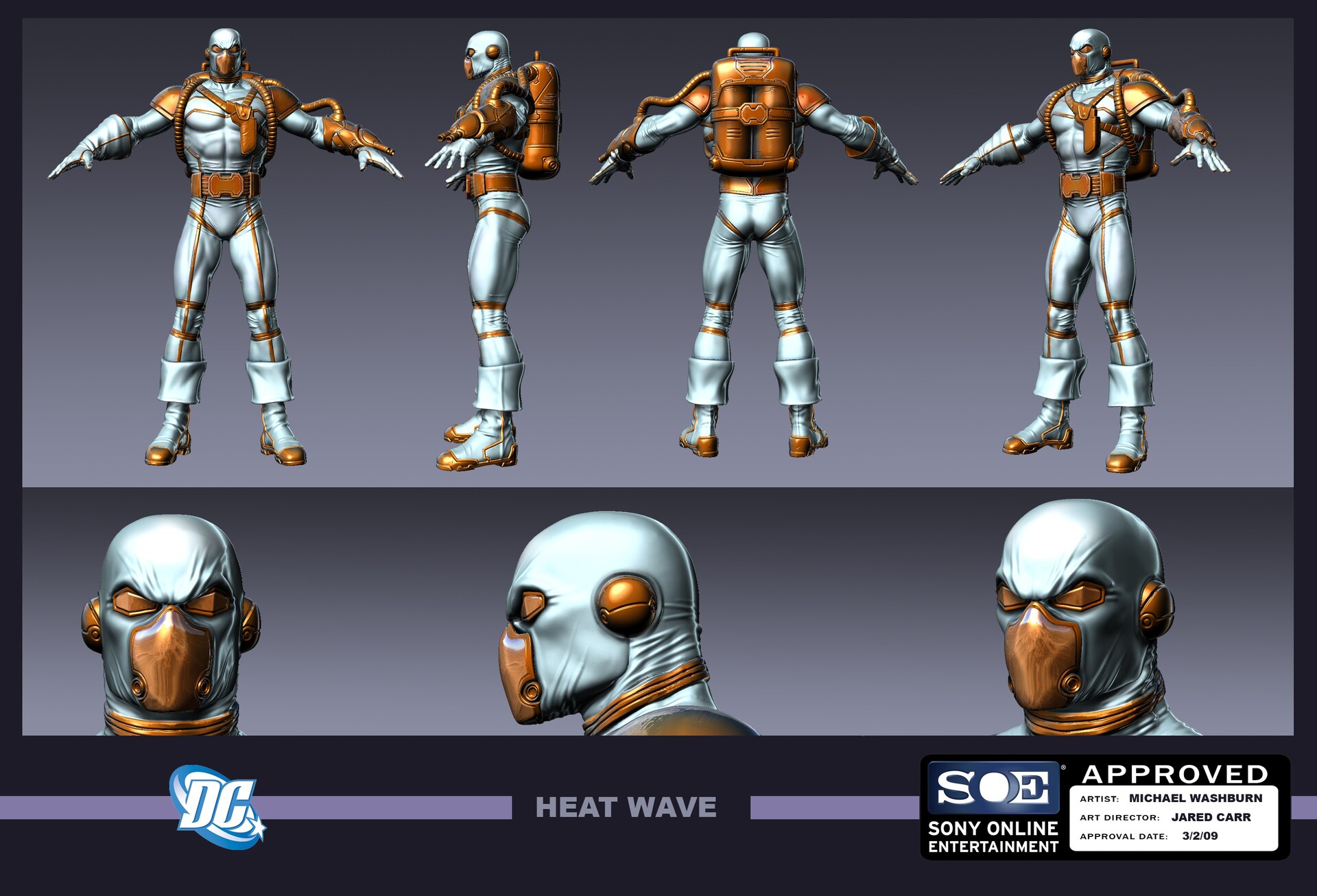This image is a detailed concept art diagram of the DC Comics video game character "Heat Wave." It features multiple angles and views of the character, providing a comprehensive visual for design purposes. At the top, there's a full-body view showcasing Heat Wave in a mainly light gray bodysuit accented with a burnt orange metallic backpack, white shoes with brown soles, and a brown belt. His mask, covering the mouth, eyes, and ears, features a mix of white and brown metallic colors.

Towards the left side of the diagram is the full front view, followed by the side view, back view, and a partially tilted view. Below these is a series of images focused on the character's head, with angles including a forward-facing, slightly left-facing, and profiles. 

The bottom of the image contains the text "Heat Wave," the DC Comics logo, and in the bottom right, the Sony Online Entertainment logo with an "Approved" stamp. Additional text includes the artist's name, Michael Washboard, Art Director Jared Carr, and the Approval Date of March 2nd, 2009. The character is presented in T-poses typical of character draft images, set against a gray background.